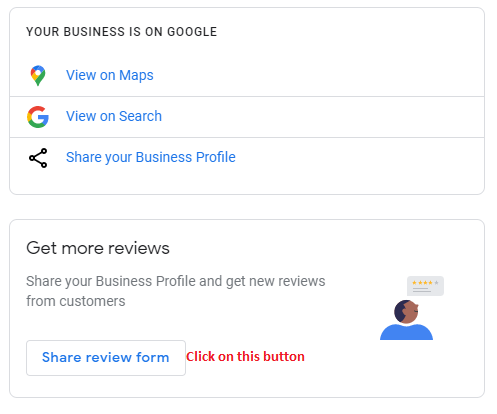The image showcases two distinct sections with a white background, each containing helpful features for managing a business profile on Google.

The upper section begins with the text "Your business is on Google" prominently positioned at the top left. Below this heading, there are three interactive options:
1. **View on Maps:** Accompanied by a Google-colored pin icon to the left, this option allows users to view their business location on Google Maps.
2. **View on Search:** Paired with the Google 'G' logo to the left, this button lets users see their business listing in Google search results.
3. **Share Your Business Profile:** Featuring an icon with three connected circles to the left, this item provides a link to share the business profile easily.

The lower section, also with a white background, is topped with the text "Get more reviews" in bold black font at the top left corner. Beneath this, it reads, "Share your business profile and get new reviews from customers." Positioned below this descriptive text is a white button labeled "Share Review Form." Adjacent to this button, in eye-catching red letters, it reads "Click on this button."

Additionally, to the right of all the text in the lower section is an illustration of a cartoon character. The character, depicted from the shoulders up, has brown skin, black hair, and wears a blue shirt. The character is looking up towards a text box displaying a four out of five-star rating, emphasizing the importance of customer reviews.